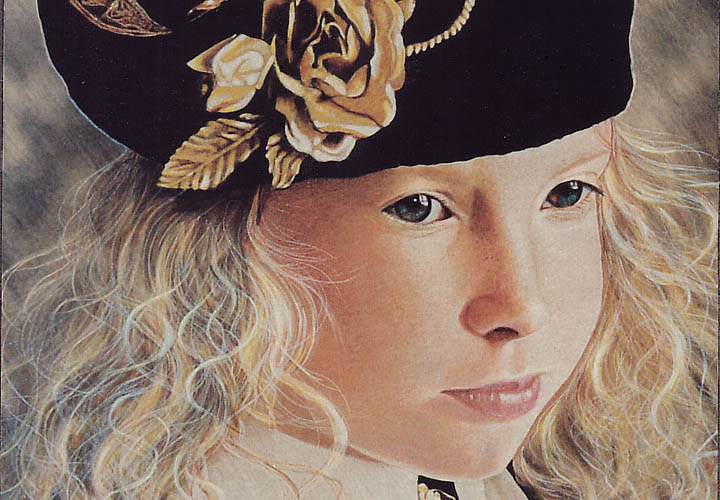Here's a detailed description of the image: 

The artwork portrays a close-up facial shot of a young girl. She is wearing a stylish black beret adorned with elegant gold flowers and delicate feathers. The girl's piercing blue eyes and her subtle, half-smiling expression are captivating. Her long, stringy blonde hair cascades down each side of her face, providing a soft contrast against the grayish background. Additionally, she is seen wearing a white beanie underneath the beret and has a collar around her neck. The girl is looking slightly off to the right, as if caught in a moment of contemplation. The color palette in the image includes hues of gold, light blonde, light brown, black, pink, and off-white. The artistic style suggests that this piece could either be a drawing or a painting, meticulously crafted to highlight her facial features, hair, and hat.